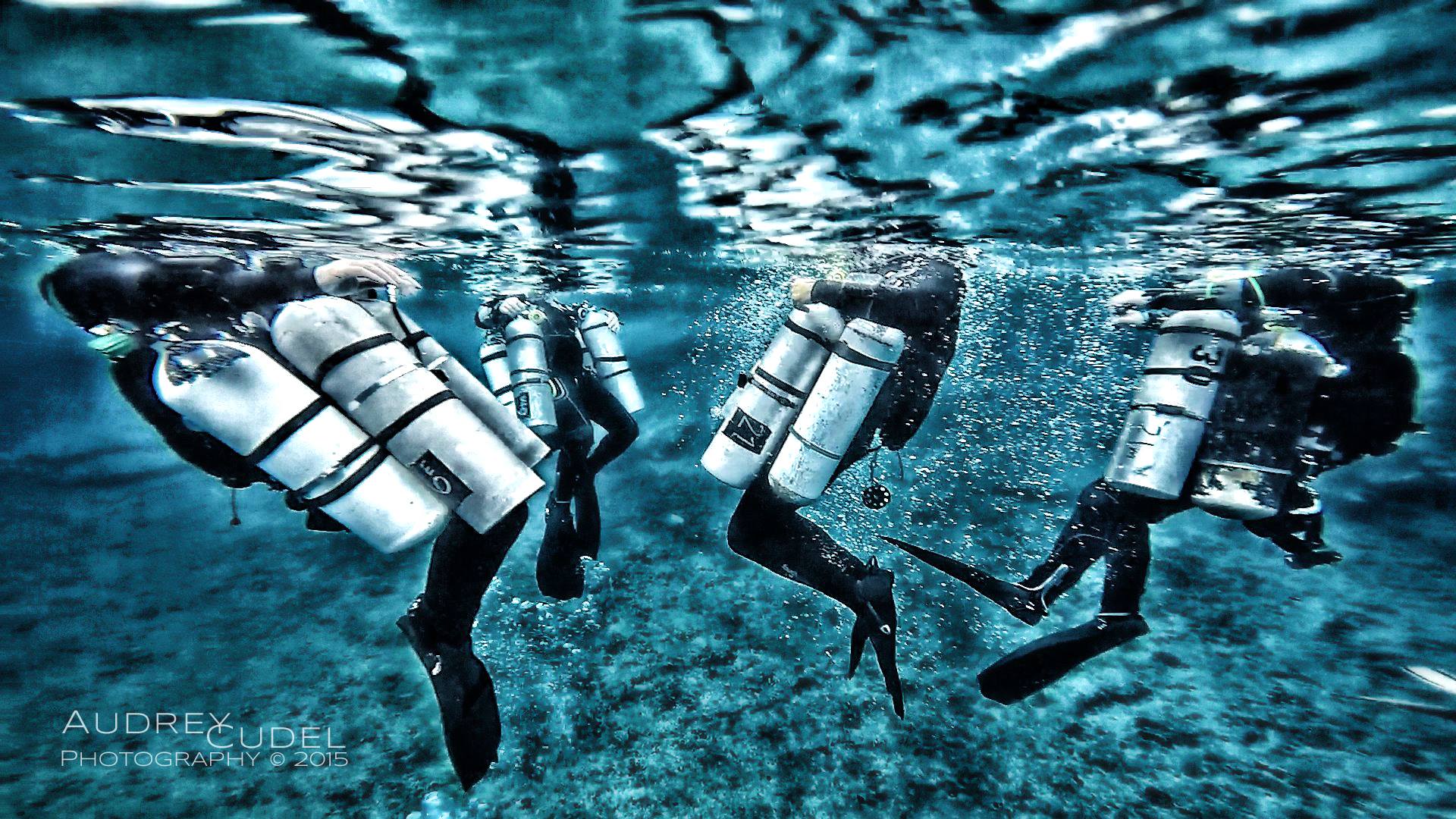The image showcases four divers partially submerged in pristine, clear blue water. Each diver is equipped with black diving suits and fins, with varying numbers of silver oxygen tanks strapped to their bodies: one diver has three tanks, another has three, a third has two, and the last has one. The water exhibits an intriguing interplay of colors, with dark and light shapes blending below the surface. The divers' heads are not visible, suggesting they are above the water. At the bottom left corner of the image, the text "Audrey Koudel, Photography, 2015" is elegantly inscribed.